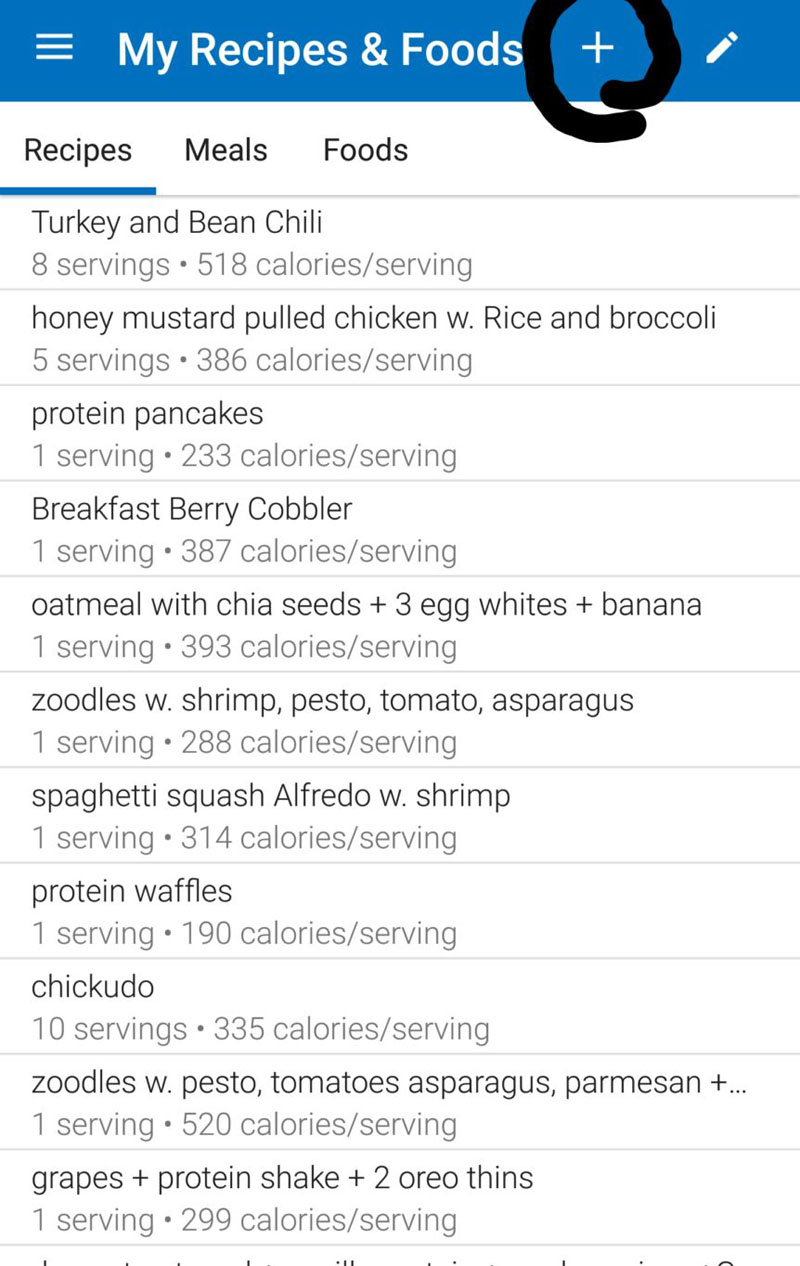In this screenshot from an app, we see an interface titled "My Recipes and Food." At the upper left corner, there is a three-line menu button, and on the upper right, a plus icon encircled in black alongside a pencil icon. Three navigation tabs are located beneath the header, labeled Recipes, Meals, and Foods. The Recipes tab is currently selected. 

The list under Recipes includes:
1. Turkey and Bean Chili
2. Honey Mustard Pulled Chicken with Rice and Broccoli
3. Protein Pancakes
4. Breakfast Berry Cobbler
5. Oatmeal with Chia Seeds plus 3 Egg Whites plus Banana
6. Zoodles with Shrimp, Pesto, Tomato, Asparagus
7. Spaghetti Squash Alfredo with Shrimp
8. Protein Waffles
9. Chickadoo
10. Zoodles with Pesto, Tomatoes, Asparagus, Parmesan
11. Grapes plus Protein Shake plus 2 Oreo Thins

Each item on the list displays the serving size and the number of calories per serving beneath its name.